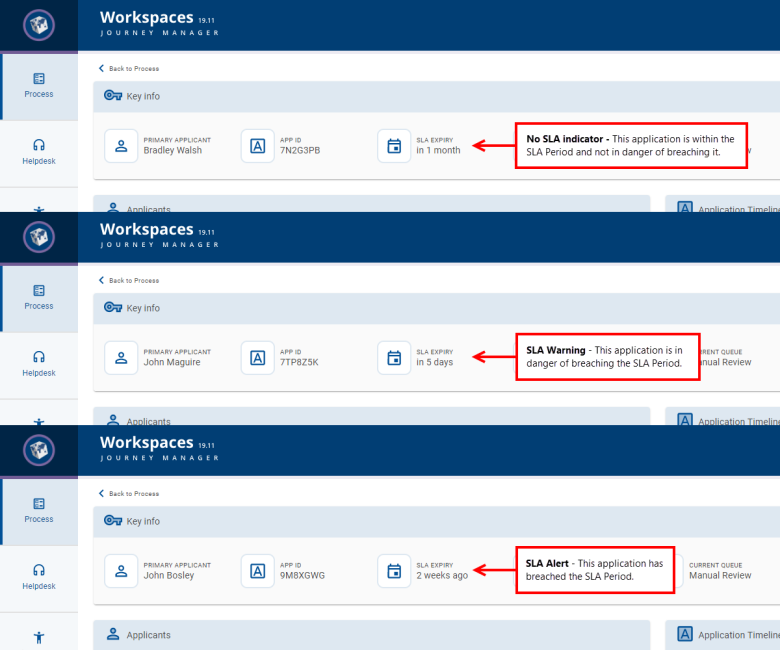This screenshot from a website displays three vertically aligned categories, each with distinct sections and elements. The topmost category features a blue thick border labeled "Workspaces" and an additional label "Journey Manager." On the left side, there is a small rectangle depicting a die within a circle. Beneath this, two tabs are visible: one labeled "Process" and another "Help Desk" accompanied by a headphones icon.

On the right, within the Content section, is a "Back to Process" label, followed by a light blue tab labeled "Key Info" with a blue key icon adjacent to it. Inside this section, three distinct boxes are present. The first box indicates that the "Primary Applicant is Bradley Walsh," accompanied by a person icon. The second box provides application details, showing "App ID: 7N2G3PV" and stating "SLA expiry in one month." The third box, labeled "No SLA Indicator," explains that "this application is within the SLA period and not in danger of breaching it."